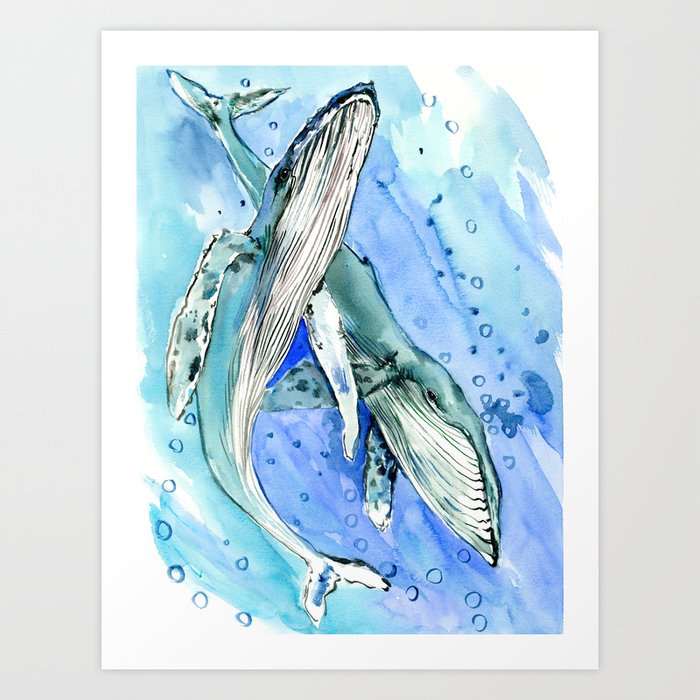This detailed watercolor painting features two orcas, or killer whales, depicted in an underwater setting. The artwork is set on a piece of white watercolor paper, which lies atop a very light gray background. The vibrant scene showcases the orcas against a backdrop of cerulean and aqua blue, with subtle hints of purple, giving the ocean its mesmerizing depth. The orca on the left is gracefully pointing upward, while the one behind it is swimming downward, their paths intertwining elegantly. Rendered with different shades of green and blue, the whales possess a greenish-gray tint and distinctive white underbellies. Black pen and ink outlines add intricate details to the whales, highlighting the artist's skill. Small bubbles are skillfully painted, enhancing the feeling of movement and life within the water. Although there is no signature or writing on the painting, the careful composition and color play speak volumes about the craftsmanship behind this captivating image.